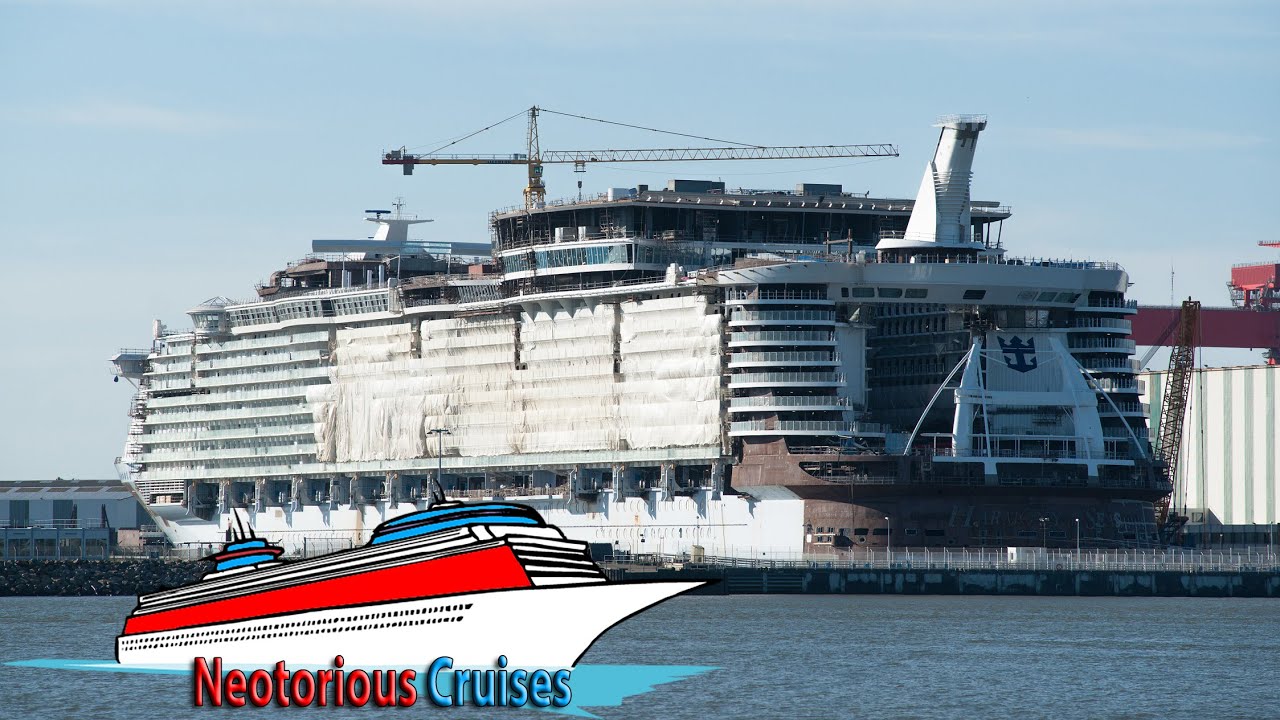The photograph captures a vast, white cruise ship docked on calm waters in what appears to be a river or bay. The background features a beautiful blue sky with a few white clouds. The ship, with multiple layers and rows of windows, shows signs of wear and tear, such as rust on the front and plastic coverings on some windows, hinting it may be undergoing repairs. At the top of the ship, there's scaffolding and a crane, possibly part of the renovation work. Along the lower back portion of the ship is a railing. In the bottom left corner of the image, there is an animated picture of a cruise ship in red, white, and blue, along with the title "Neo-Torreus Cruises," serving as a distinct logo for the vessel. The dock and surrounding structures further emphasize the ship's immense size and current stationary state.